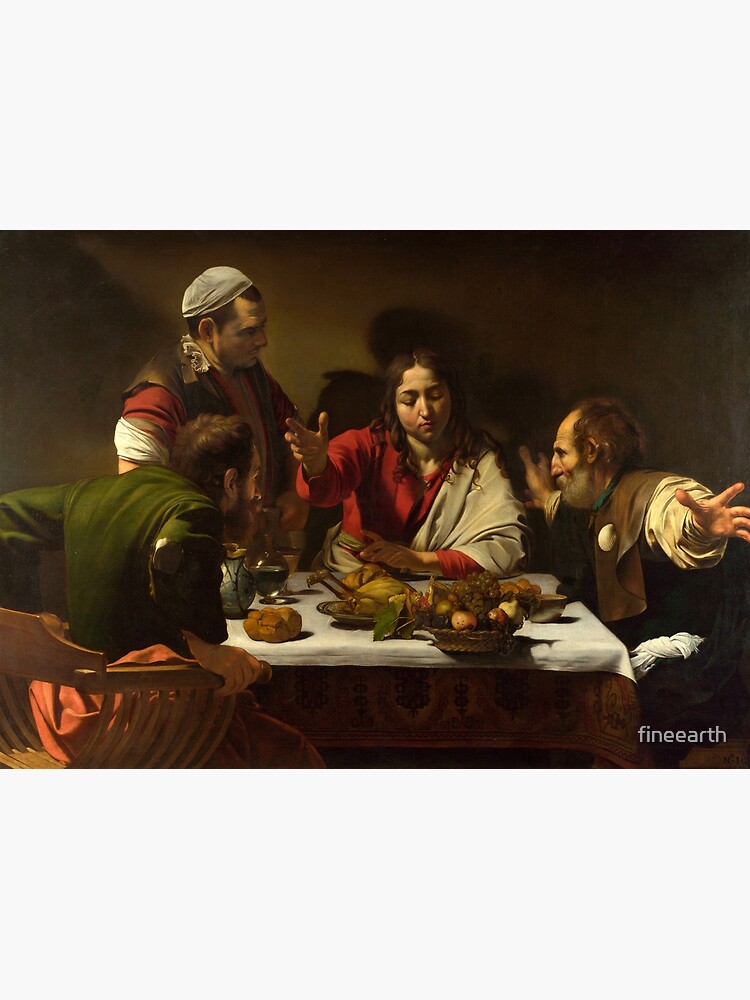This detailed painting, labeled "Vintage Wall Art" in white text in the bottom right corner, is a rectangular image oriented horizontally. It depicts a group of four Caucasian individuals dressed in old-fashioned garments that suggest a historical or vintage setting. Three of the people, two men and a woman, are seated around a small, white-clothed dinner table bearing fruits, including grapes and peaches, as well as a cooked chicken with its legs up and a loaf of bread. The man to the left, dressed in a green shirt, has his back to the viewer. The elderly man to the right, identifiable by his white beard and wearing a brown tunic over a white shirt, has his arms spread wide. At the head of the table sits a woman with long black hair, clad in a red and white shirt, eyes closed and right hand extended as if gesturing during a discussion. Standing next to her is another man in a white beanie. The group appears engaged in an intense conversation, with some tension suggested among them, further adding to the antiquated and evocative atmosphere of the painting. The dominant colors in the artwork are red and brown, complemented by touches of white, green, gray, and black, enhancing the overall rustic and historic feel of the scene.